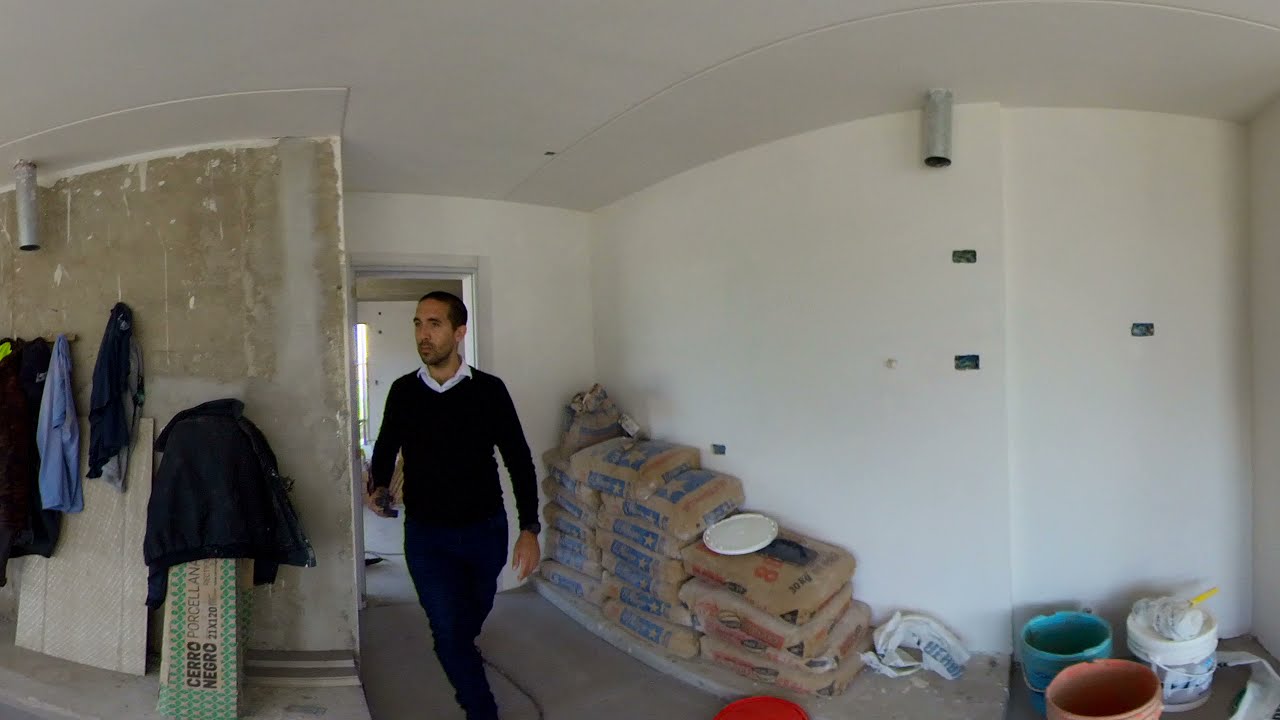The image depicts a room inside a building undergoing construction. Most walls are white plastered, but an unfinished wall is visible on the left. The floor shows some scattered tiles yet to be placed. A man, appearing to be around age 40 with short black hair and a scraggly mustache-beard combination, stands in the middle of the room looking to the left. He has a darker skin complexion and wears black pants paired with a black sweater over a white collared shirt. A door just left of center behind him lets in natural daylight, illuminating the room clearly. On the right side of the image, bags of concrete are stacked, packaged in brown paper. In the bottom right corner, several buckets are visible, one green, one white, and one orange. Articles of clothing hang on the unfinished wall to the left. Overall, the image is bright and sharply detailed, highlighting the active construction environment.